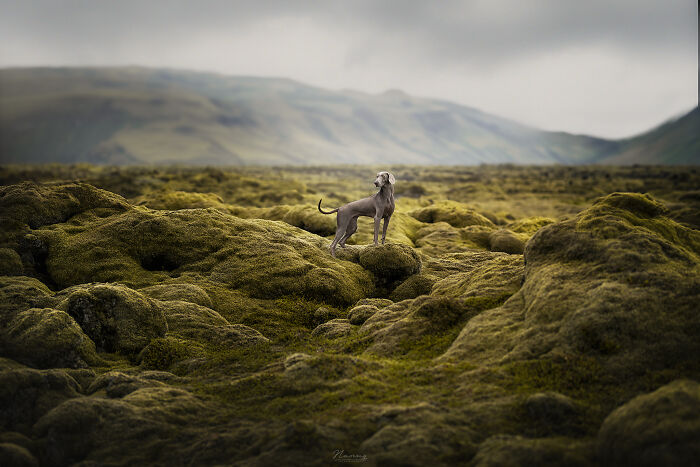In the image, a tall, long, gray hound stands atop a moss-covered boulder in the middle of a rocky and uneven plain, which stretches out as far as the eye can see, covered with lumps of boulders beneath the grassy surface. The dog’s body is oriented to the right, but its head turns to the left, allowing a view of its light gray, almost shaved short hair, long tail, and floppy ears. The two front legs rest slightly higher on a raised rock compared to its back legs, and the tail curves to the left side of its body. The sky above is thick with dark rain clouds, casting a gray hue over the landscape. In the background, hilly mountain ranges appear faint and washed out, partially obscured by low-hanging fog and cloud cover, and suffused with green from the grassy surface. Despite the overcast skies, a beam of sunlight breaks through, illuminating the hound’s back and head as it stands alone in this serene and desolate expanse.